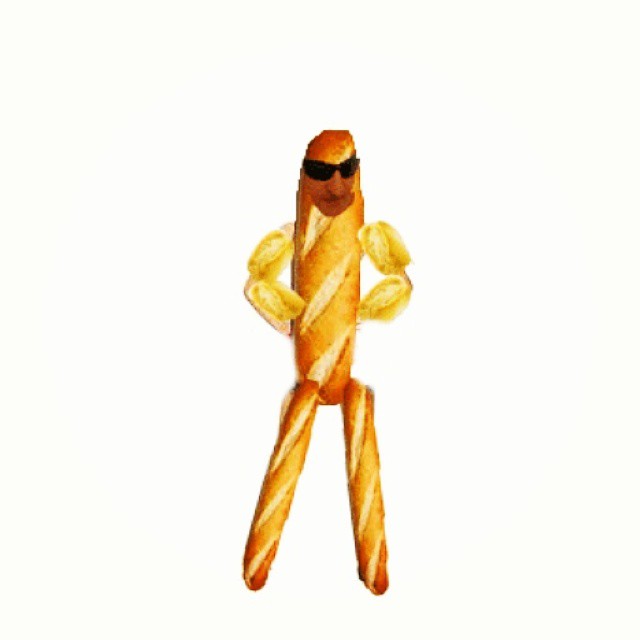The image depicts a whimsical figure assembled from various types of bread, resembling a stick person. The figure stands upright against a mostly white, slightly gray background. Its body is formed from a thicker, longer piece of bread, while the legs are represented by two long, thin breadsticks. The arms, portrayed by smaller, bent pieces of bread, are folded across the midsection, giving the impression of 'bread hands' holding the body's center. A real human face, edited onto the top, is cropped at the hairline and features black sunglasses, with no ears or other facial details visible. The overall color scheme of the bread components ranges from beige to tan, indicating well-baked bread.